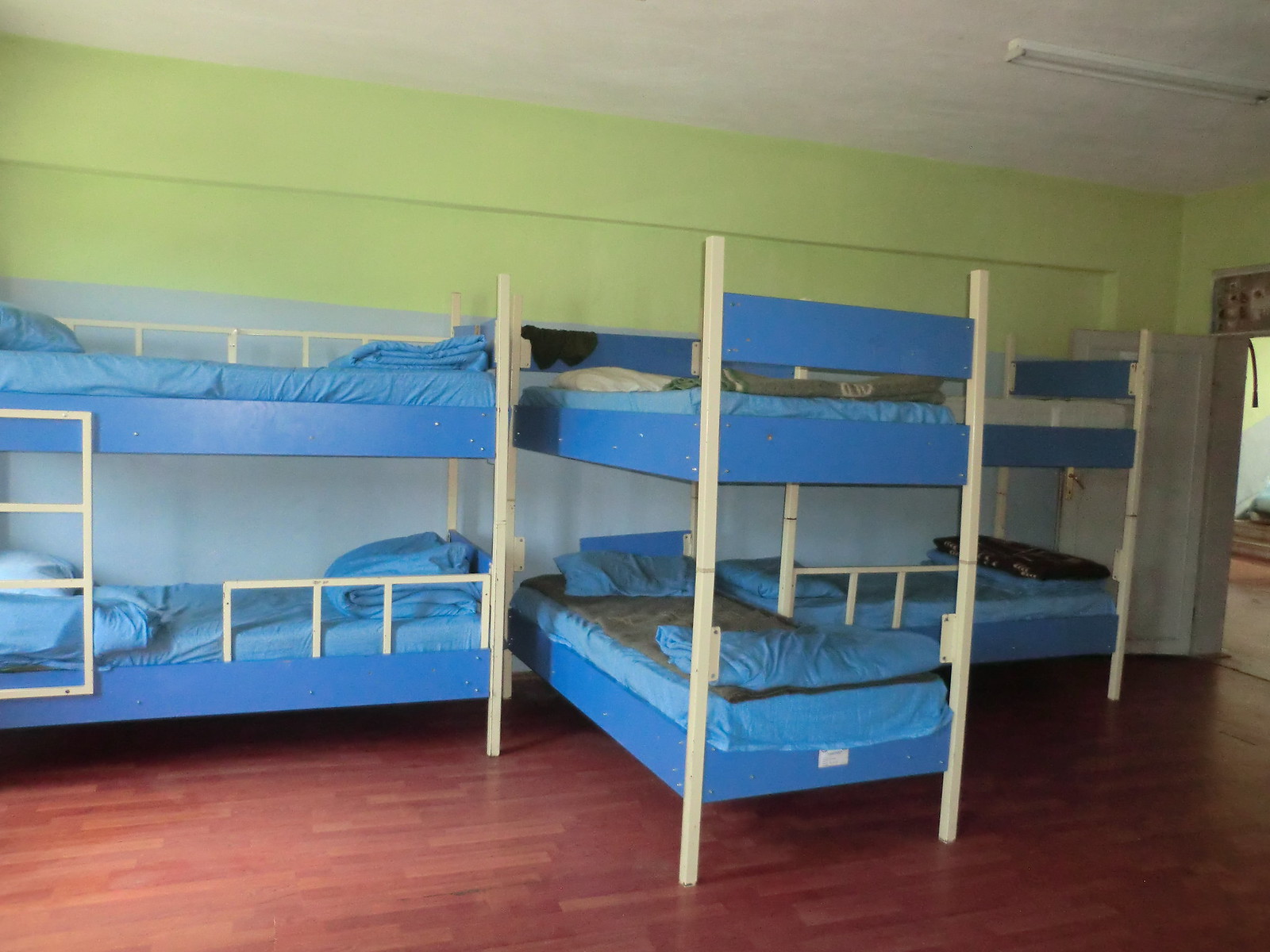In the photograph of a dormitory room, there are three interconnected bunk bed sets positioned in a T-formation. Two of the bunk beds are placed horizontally while the third one is positioned vertically in the center. The bunk bed frames are primarily dark blue with corner support beams featuring a light woodish color. The bedding includes lighter blue sheets and pillows, with some beds having unique blankets—one with an army green blanket and another with a black blanket. The beds occupy most of the room's space and have a clear hierarchical order, with an extra black cushion on the middle vertical bed and some items like shorts on the upper frames.

The room is painted with a lime green wall extending two-thirds up, topped with a light green shade. The floor is a dark cherry wood linoleum, polished to a sheen. A unique feature of the room is an indentation in the wall that creates a slight alcove. There’s an open white door on the right-hand side, adorned with a decorative element resembling two dog heads above it. A hanging ceiling light with two fluorescent bulbs illuminates the room from above. The ceiling itself is a white cream color, smooth and reflective, enhancing the natural light that streams in. Additionally, there is some kind of piping visible on the adjacent wall, adding to the room's utilitarian feel.